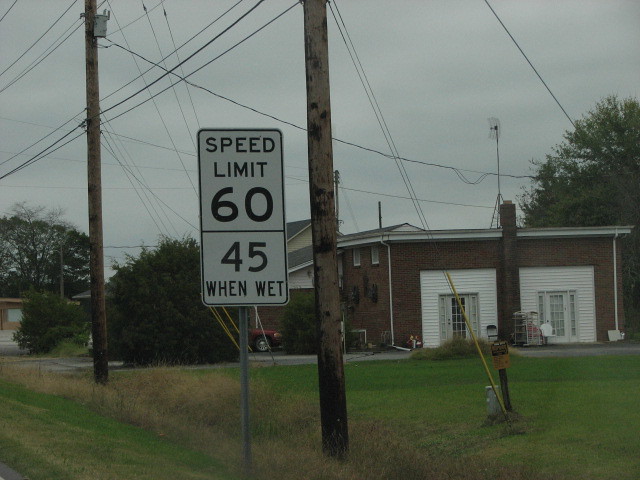In this color photograph taken on a cloudy, overcast day, the focal point is a speed limit sign centrally placed towards the left. The sign is on a gray metal pole and features black lettering on a white background, indicating "Speed Limit 60" and "45 When Wet" beneath it. Surrounding the sign is a scene of dry, unkempt grass. 

To the left and right of the speed limit sign are two electrical poles. The nearest pole on the left is a typical brown wooden telephone pole. The pole on the right, set in a ditch with yellow-covered anchor cables securing it to the ground, is also wooden. Numerous wires stretch between these poles and a nearby brick house. 

Behind the speed limit sign, setting part of the backdrop, is the brick house featuring a flat roof and two entrances with blue and green doors. There are patches of white siding, a chimney, and an antenna on the roof. Another house with only its roof peaks visible stands in the background. Adding to the predominantly residential scene are trees and bushes, contributing to the greenery amidst the overcast sky.